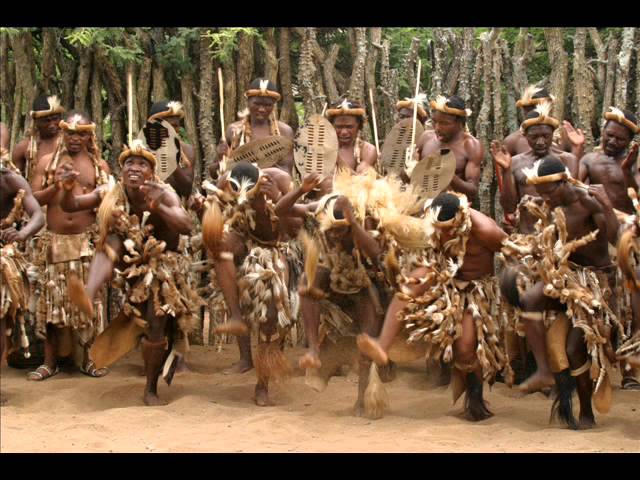The image depicts a vibrant tribal dance scene featuring between 10 to 15 darker-skinned men, likely of African or perhaps Hawaiian descent, dressed in traditional attire. They perform against a backdrop of sandy terrain with palm trees in the distance. In two distinct rows, the front row of men raises their right legs as if stomping on the ground, energetically bent over in a spirited dance. These performers are shirtless, wearing thin skirts adorned with feathers and woolly strands, and brown headbands accentuated with feathers protruding from the front. Some men also have woolly necklaces. Behind the dancers, a second row of men appears to be playing oval-shaped percussion instruments with sticks, and some are clapping, contributing to the rhythmic music that accompanies the dance. The combination of dynamic movement, traditional costumes, and lively instrumentation captures the essence of a rich cultural performance.